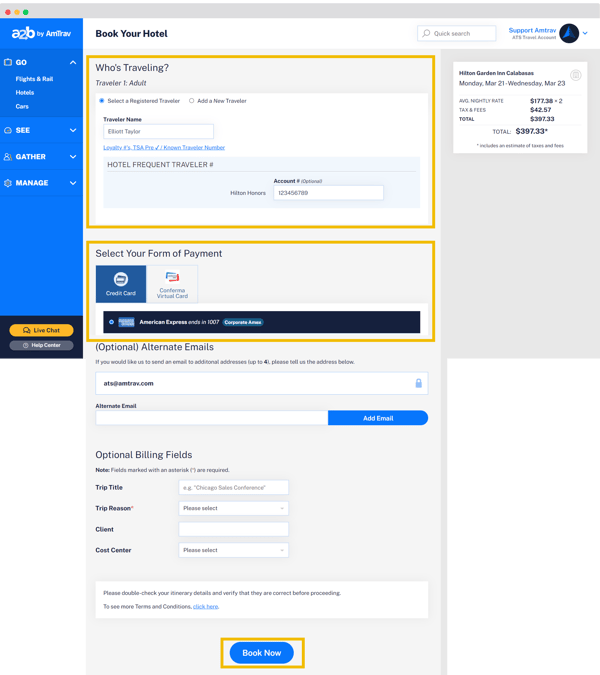A screenshot features a booking interface with a blue rectangle displaying "A2B" in white text, by what appears to be "Amtra" (A-M-T-R-A), with the letters "A-N-T" capitalized. The screen prompts users to "Book Your Hotel" and includes a search bar. There's a dropdown asking "Who's Traveling?" where various options such as "Traveler", "Adult", and "Traveler audit" can be selected. Users can choose their form of payment from two options: a blue square labeled "Credit Card" and a white square labeled "Conference Virtual Card." Additional optional fields for alternate emails and billing details are provided. The interface also includes input bars for "Trip Title," "Trip Reason," "Client," and "Cost Carrier."